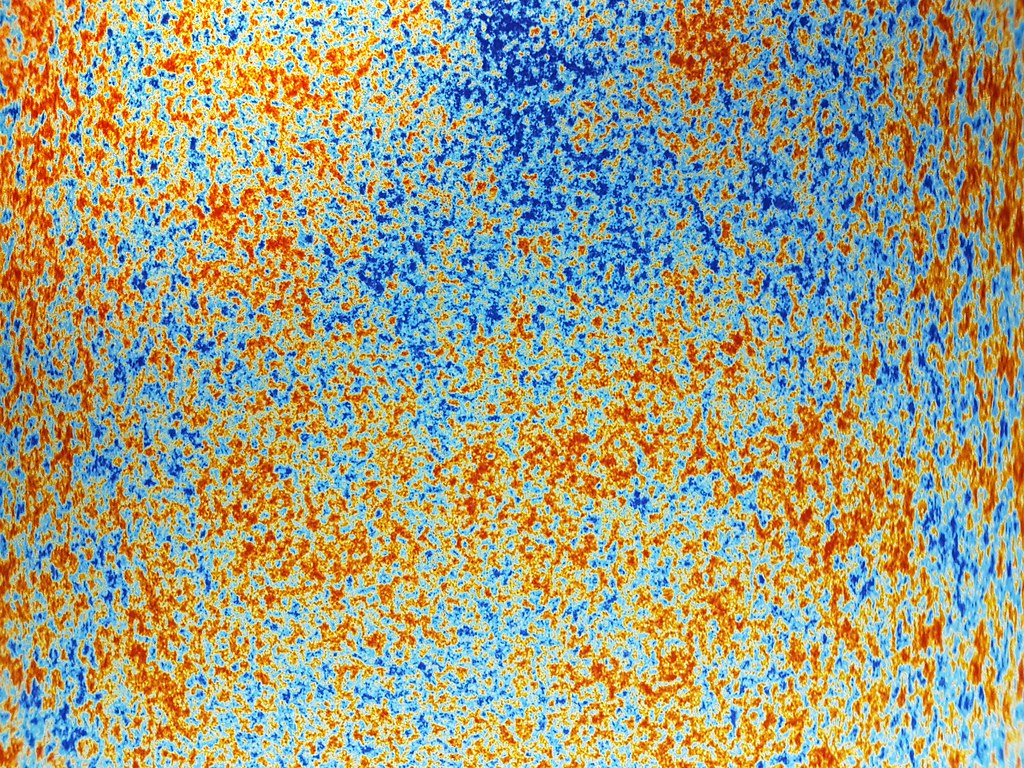This image is an abstract illustration resembling a thermal heat map, featuring a rough, speckled pattern composed of contrasting colors. The pattern includes clusters of red, yellow, blue, and light blue, which are randomly scattered yet fairly evenly distributed across the canvas. These clusters create a detailed, speckled effect that mimics the appearance of rust or splashes of paint. The colors vary in intensity, with gradients ranging from light to dark blue and from light to dark orange. Despite the mixed appearance, the individual spots of color remain distinct, collectively forming a complex and textured visual without any specific image or silhouette.